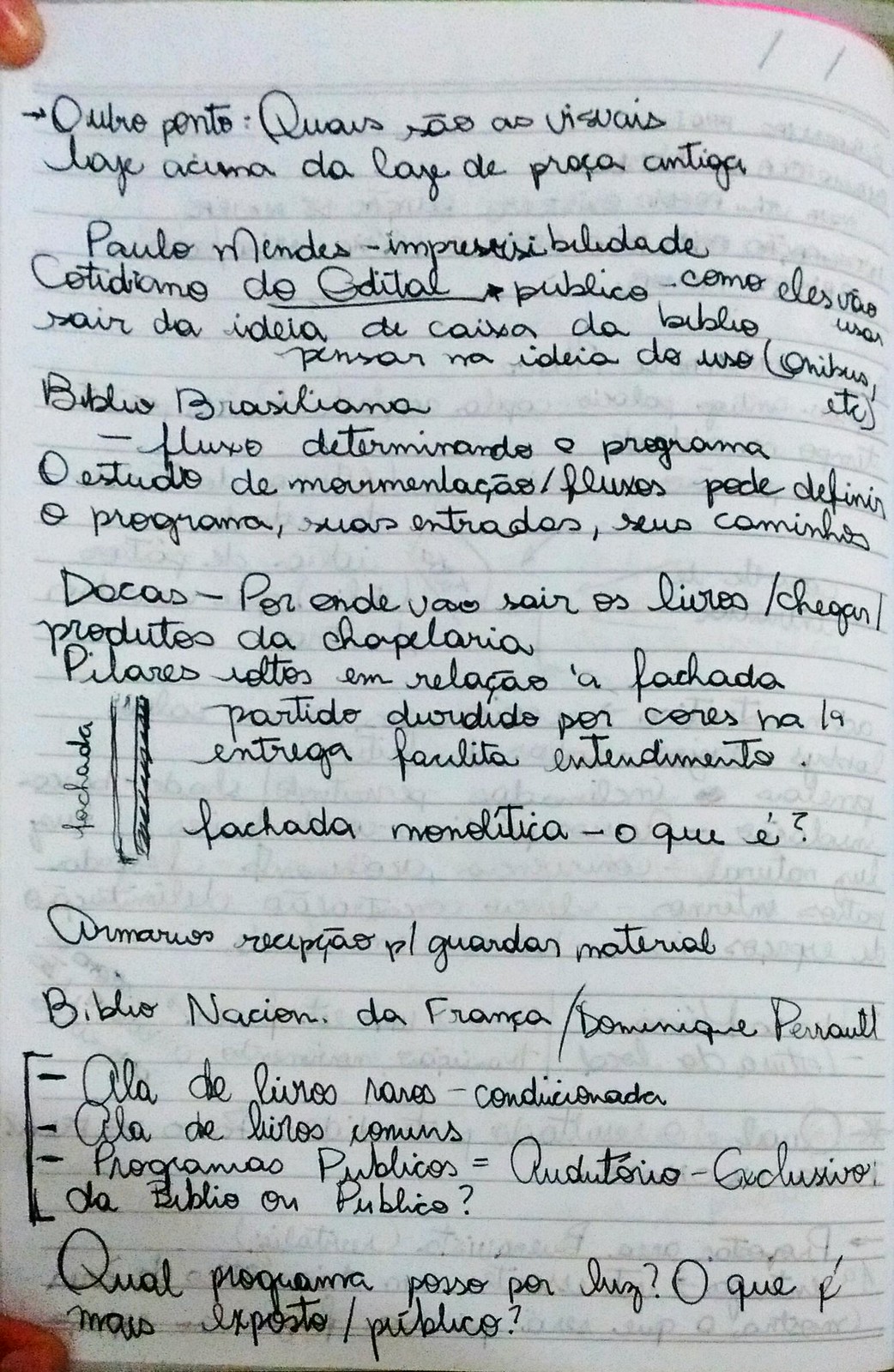The photograph depicts a page from a lined notebook filled with handwritten text in black ink. The text, primarily in Spanish, encompasses the entire page, featuring both cursive and block print handwriting. Notable elements include the words "Centrodome de Capital" and "Qual Programma" prominently mentioned on the page. There is clarity in the script, indicating legible handwriting. The paper shows signs of writing on the reverse side, visible through the thin white paper. Additionally, a black bracket on the left-hand side encloses three bulleted points. The page is held open by fingers at both the upper left and lower left corners. A pink line borders the top of the paper, with the rest of the lines on the paper appearing in black or gray. The overall content includes a few varied words like "Abre," "Pento," "Palo," "Mendez," "Biblias," "Rosalina," and others, interspersed with a couple of simple line diagrams accenting the left margin.